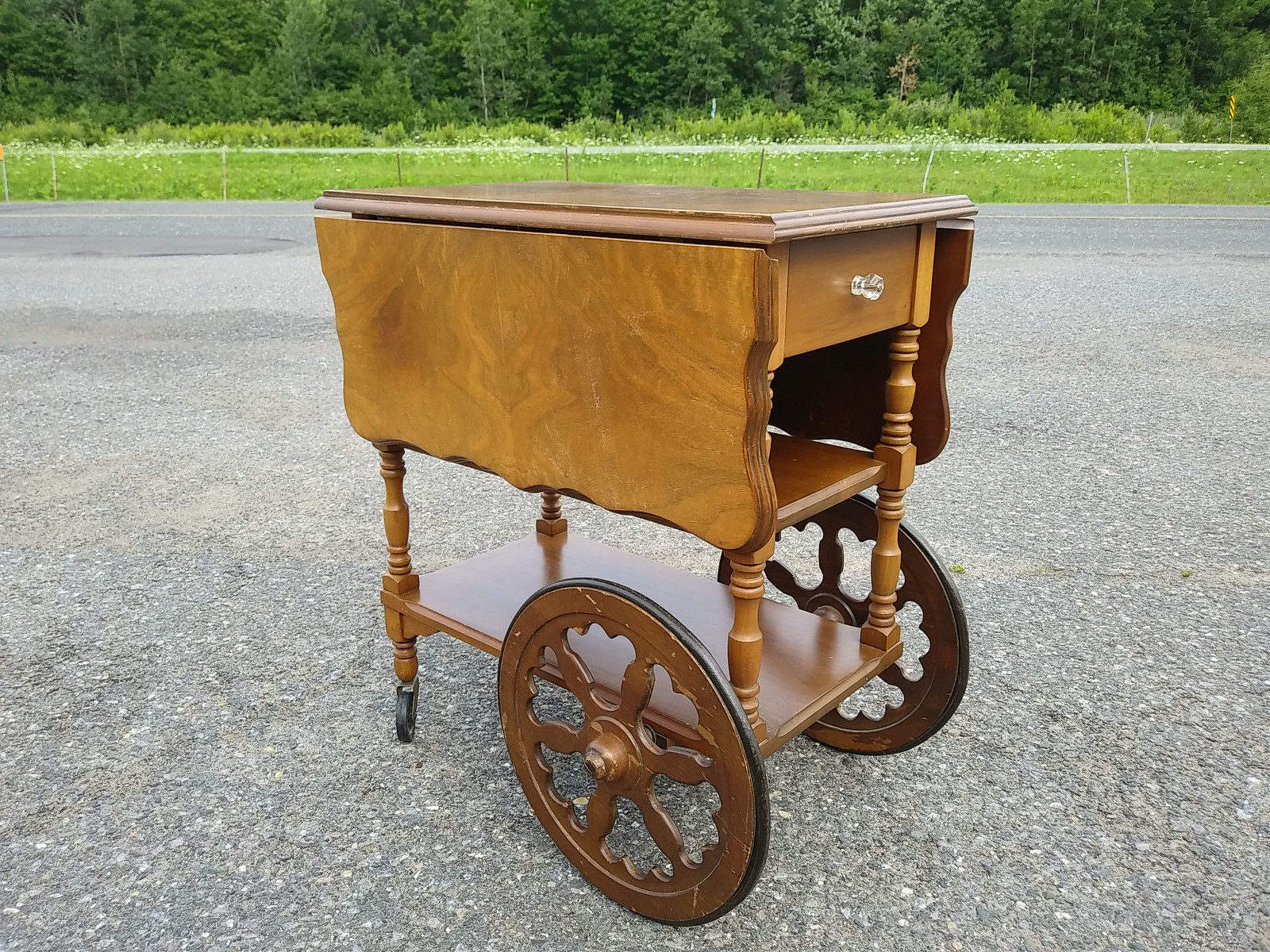The image depicts a vintage wooden cart with a well-crafted design, positioned diagonally on a gray asphalt surface. The cart features a single pull-out drawer with a clear crystal-looking knob. Its tabletop includes collapsible drop leaf sides. The cart is equipped with four wheels: two large wooden wheels with a black tread on one side, which are fixed, and two smaller, rotating wheels on the other side. Surrounding the cart, there is a picturesque outdoor setting with green shrubbery, grass, and darker green trees, indicating an outdoor parking lot or driveway taken during daytime. The cart's intricate woodwork and functionality make it the focal point of the photo.